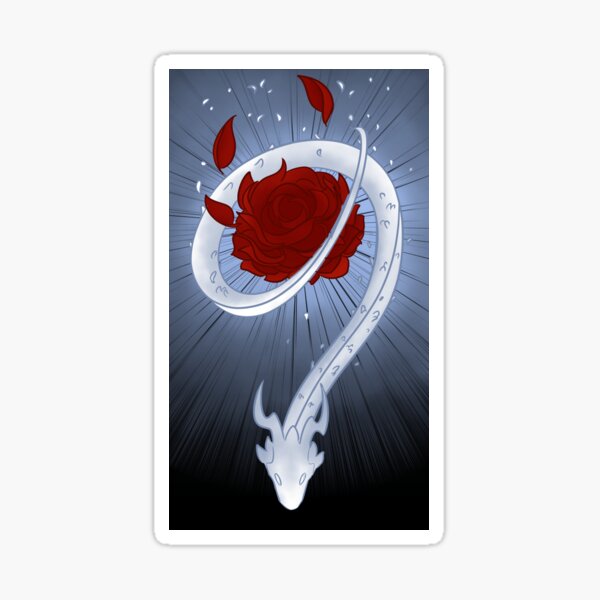This detailed drawing of a card features a surreal and dramatic illustration. The card, in portrait orientation, has a white border that frames a gradient background transitioning from light gray at the top to nearly black at the bottom. Central to the artwork is a striking image of a light blue and white snake, its body adorned with intricate scale markings. The snake, with a snub nose and horn-like protrusions on its head, gracefully encircles a vibrant red rose. Some petals of the rose have fallen and appear to float around the flower. The snake's tail starts in the upper right corner, wraps counterclockwise around the rose, and then curves back clockwise, directing the viewer’s eye down to the center where the snake's head points downward. The illustration conveys a sense of mythical beauty, emphasizing the contrast between the delicate rose petals and the sinuous, dragon-like creature.